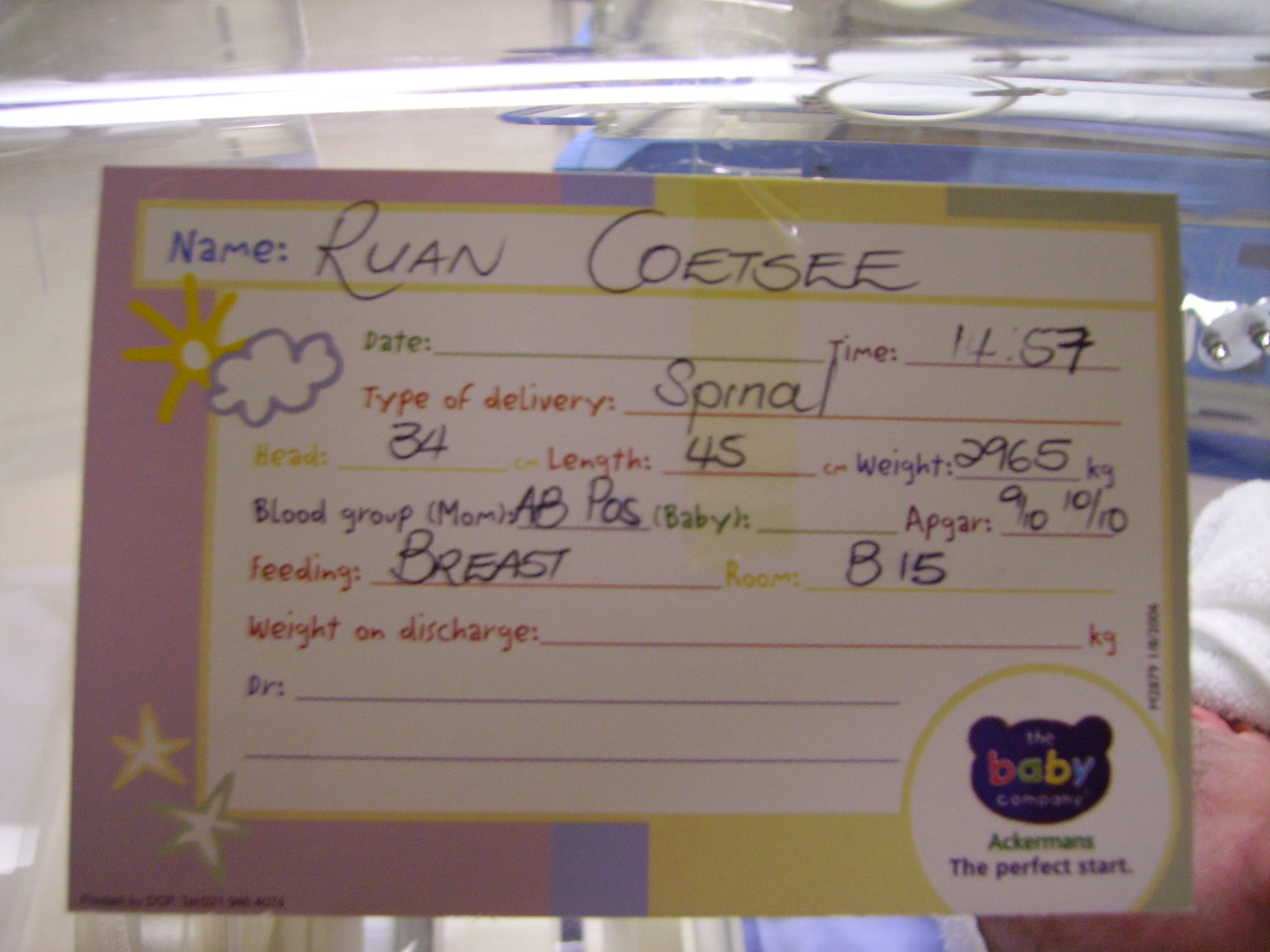This photograph features a detailed card from The Baby Company, titled "Ackermann's The Perfect Start," indicating the birth of a baby named Ruan Coetzee. The card, adorned with pastel shades of purple, blue, yellow, and green, along with stars and clouds around the edges, is likely taped to the outside of a baby incubator or resting area, though the background is obscured. At the top of the card, it lists key details: 

- **Name:** Ruan Coetzee 
- **Time:** 14:57 
- **Type of Delivery:** Spinal
- **Head Circumference:** 34 centimeters 
- **Length:** 45 centimeters 
- **Weight:** 2.965 kilograms (2,965 grams)
- **Blood Group:** AB positive (Mother's)
- **APGAR Score:** 9/10 and 10/10 
- **Feeding:** Breast  
- **Room:** B15

There are also sections for the date, weight on discharge in kilograms, and the doctor’s name, which remain unfilled.